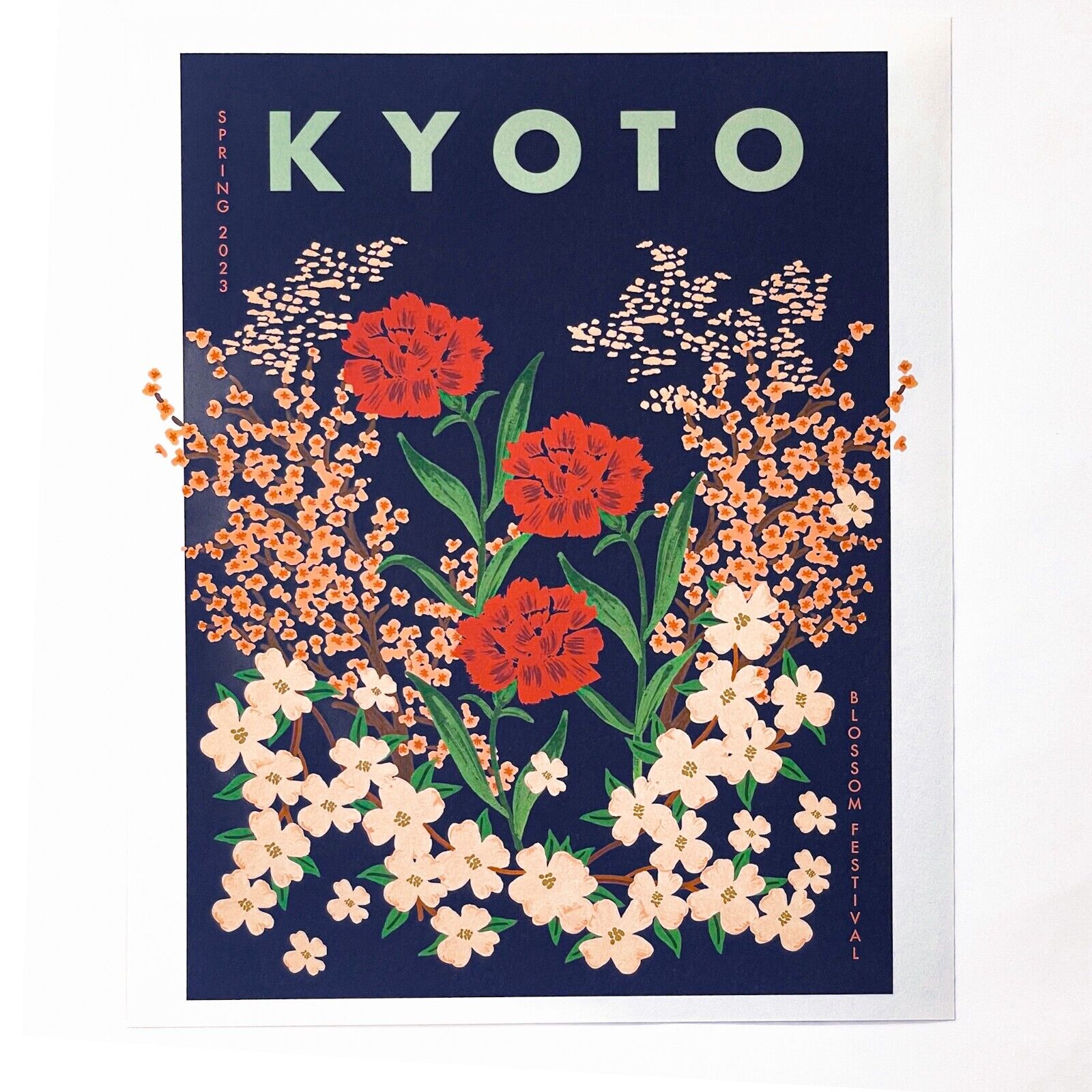This image is a vibrant poster for the Kyoto Blossom Festival from Spring 2023. Dominating the poster is a deep blue background, framed by a thin white border, giving it a polished look as if it were mounted on a light gray wall. At the top in large block letters, "Kyoto" is prominently displayed in a pale green or teal color. Just below, a stunning array of flowers captures the eye; bright red blooms, delicate white flowers with yellow centers, small clusters of orange flowers with darker orange centers, and a sprinkling of light pink and off-white blossoms can be seen, all supported by green stems and intertwined with brown branches. In smaller font, the words "Spring 2023" run vertically in a pinkish-red hue on the upper left side of the poster, beside "Kyoto." Completing the design, the text "Blossom Festival" is elegantly placed in the bottom right corner, also spanning downwards.